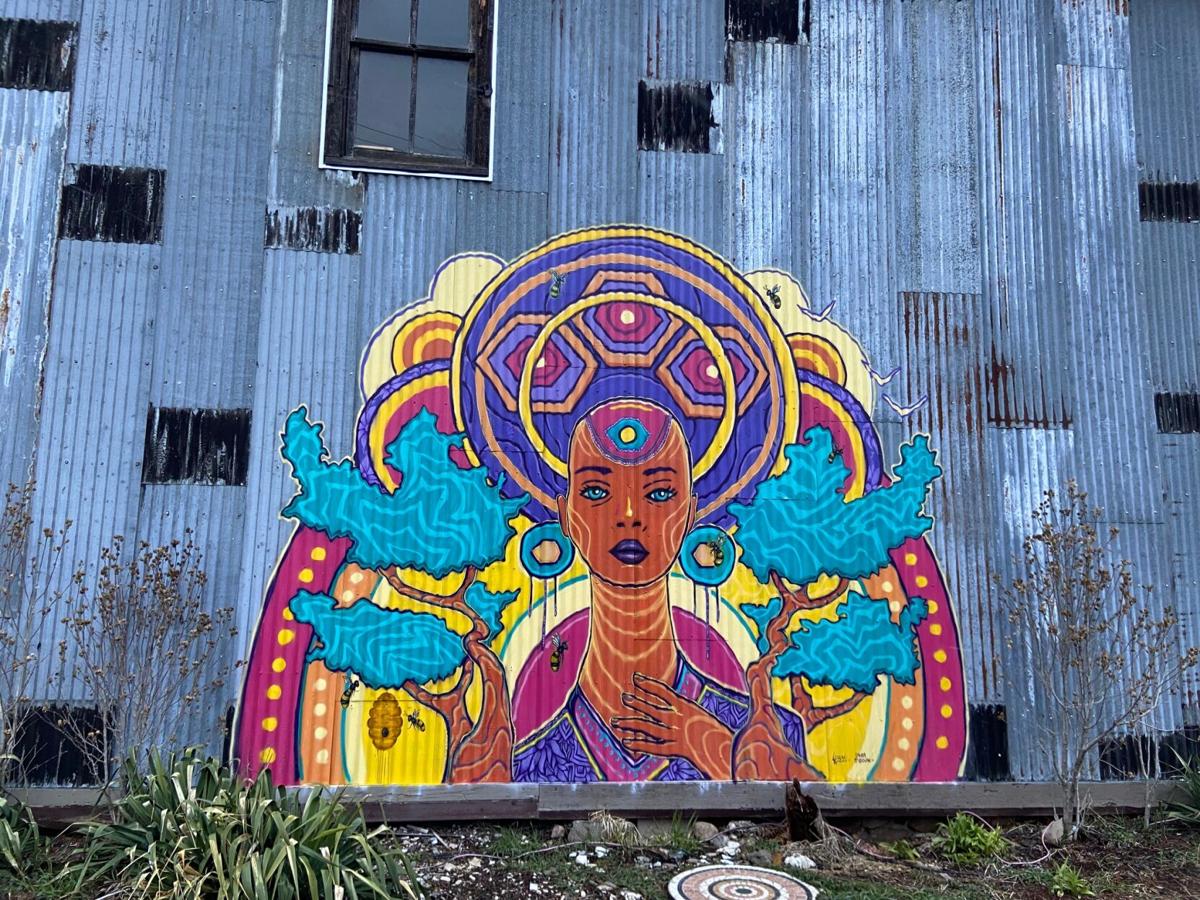The image depicts a vibrant, outdoor mural painted on a blue, possibly wooden, wall with gaps and signs of dirt and moss. The mural showcases a dark-skinned African woman adorned with elaborate headwear featuring intricate patterns in purple, blue, and yellow. The woman, who resembles an African goddess, has a long neck and blue earrings, and her left hand gently touches her neck. Surrounding her head is a series of decorative circles in purple, gold, and yellow. Flanking the mural are brown trees with eye-catching turquoise or blue leaves. The background above the mural reveals an old, unused window, while the foreground displays a circular mosaic tile pattern amidst dry grass, ferns, and scattered shrubbery. Additionally, there are bees or wasps flying around the woman, adding life to the scene.